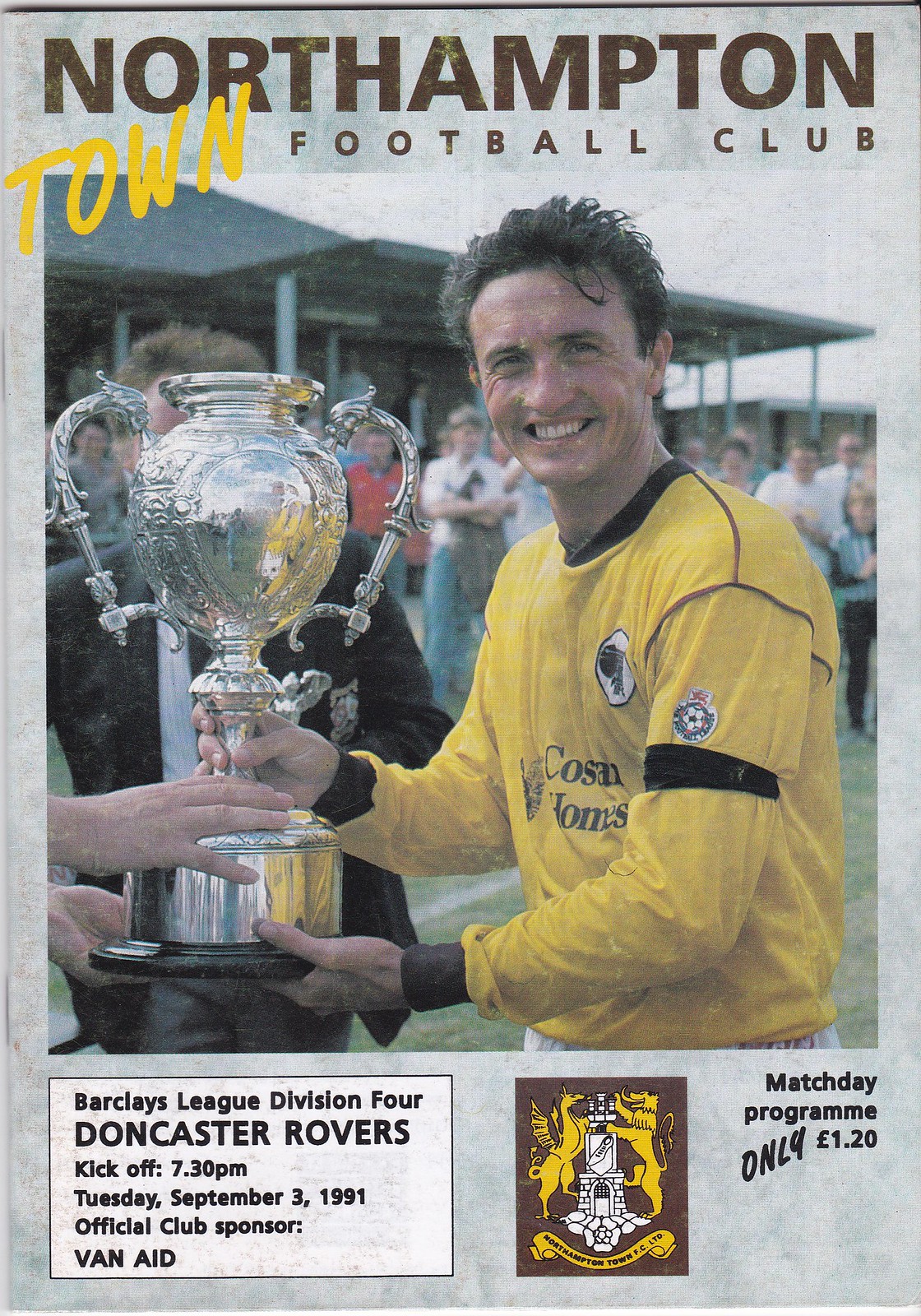The cover of the Northampton Town Football Club match-day program features a predominantly grey marble background. At the top, 'Northampton Football Club' is prominently displayed in brown text, with the word 'town' artistically written in yellow just to the left. Dominating the center of the cover is a photograph of a soccer player wearing a long-sleeved, yellow jersey with a black collar and black wrist details. The player is facing left but looks directly at the camera, smiling as he holds a large silver trophy with a round black base handed to him from off-screen. He appears to be sweating, adding to the intensity of the moment. Below the photograph, black text provides crucial match details: 'Barclays League Division 4 Doncaster Rovers kickoff 7.30pm Tuesday, September 3, 1991 Official Club Sponsor Van Aid.' An insignia of the Northampton Town Football Club is also visible. The program is advertised as a bargain, costing only £1.20 or the equivalent in euros.